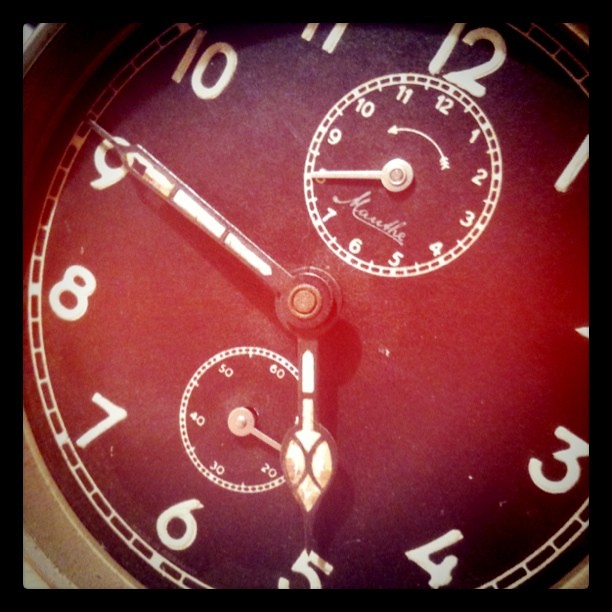A close-up photograph of a Mauthe watch, displaying a partial yet detailed view of its intricately designed face. The off-center composition captures the classic Arabic numerals for hours, although some of the outer edges are cut off. Two small subdials are prominently visible in the central area of the watch face. The upper subdial features the hour markers from 1 to 12, while the lower subdial appears to track the passing seconds. The name of the watchmaker, "Mauthe," is subtly inscribed, adding a touch of elegance and authenticity to this timeless piece.